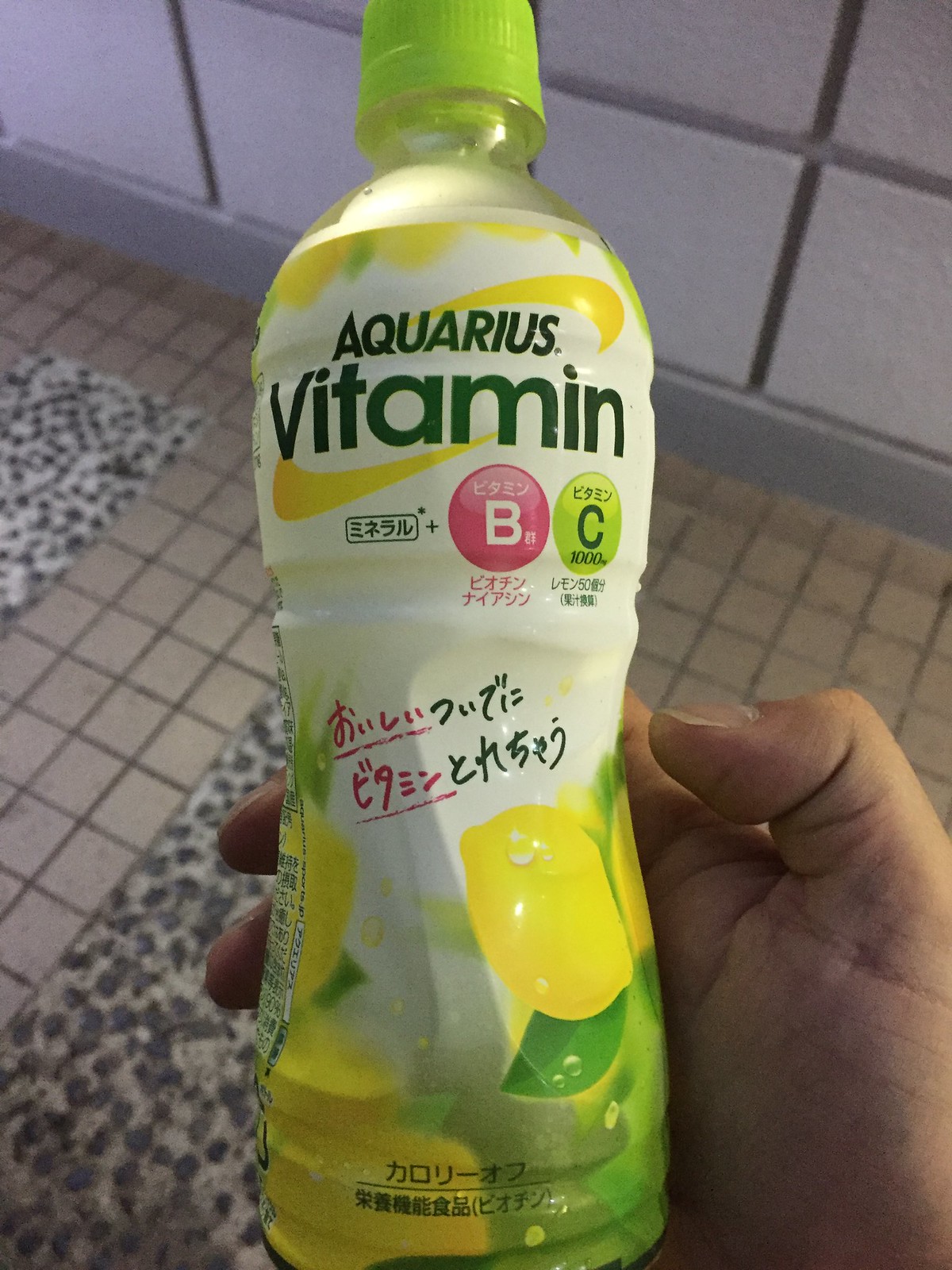The image showcases a hand holding a plastic drink bottle adorned with extensive Japanese lettering. Topped with a lemon-yellow lid, the bottle is clear with a wrapped plastic sleeve that prominently displays the brand name "Aquarius Vitamin." The sleeve features the letters "B" and "C," suggesting the inclusion of vitamins B12 and C, with the numeral "1000" listed under the letter C, likely indicating the milligram content of vitamin C. The label also depicts a vibrant lemon and a lemon leaf, hinting at the flavor or key ingredients of the beverage, which appears to be lemon-flavored water or vitamin-enriched water rather than juice. In the background, there is a dingy gray tile floor cluttered with black and white spotted mats, adding a domestic and somewhat gritty context to the scene.